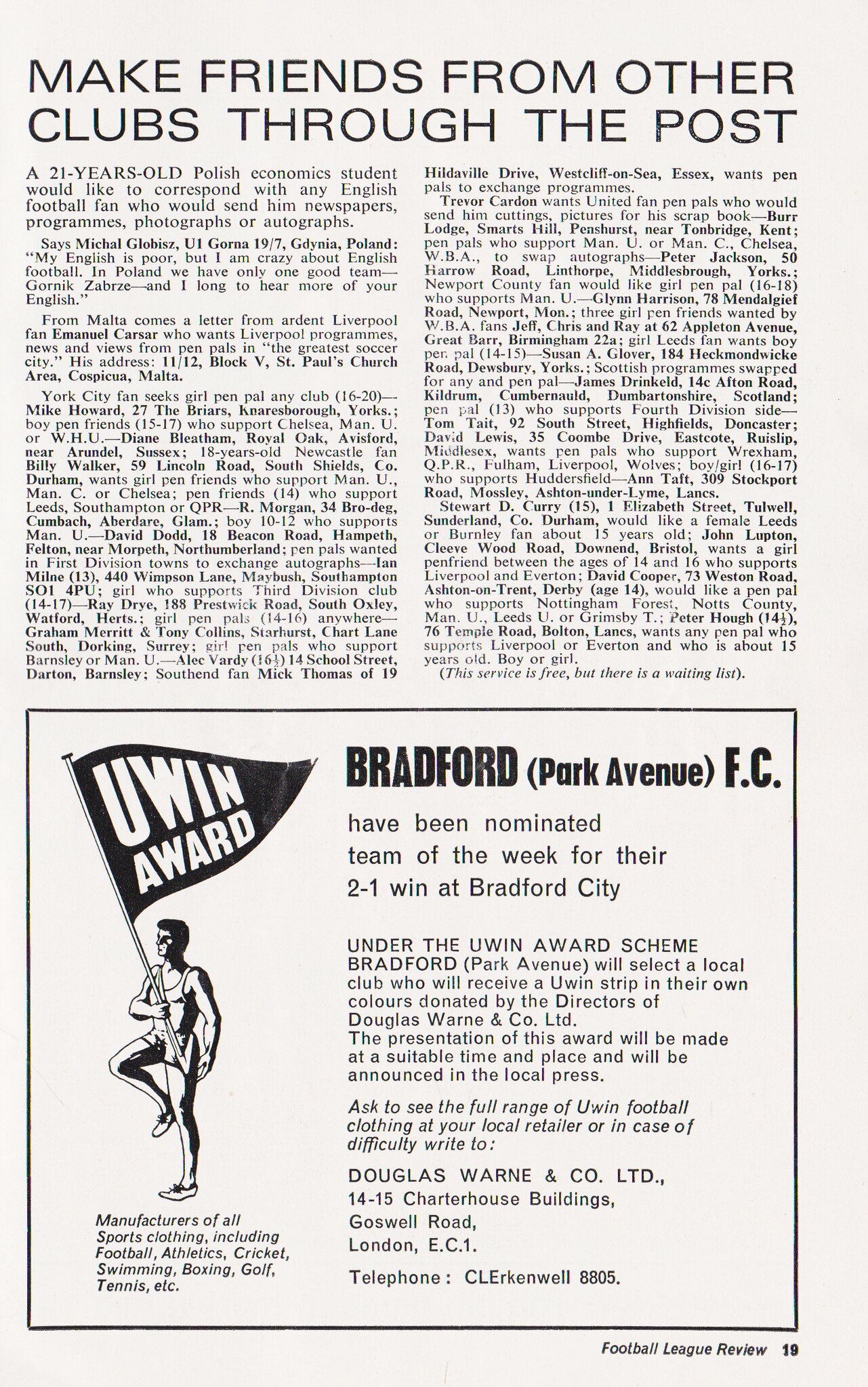The image depicts page 19 of the Football League Review, featuring a blend of a lengthy list of names and ages, articles, and advertisements. At the top of the page, under the headline "Make friends from other clubs through the post," there is a detailed announcement: a 21-year-old Polish economics student named Michael Globicz from U.I. Gorna, 19-7, Gdynia, Poland, seeks to correspond with any English football fans who can send him newspapers, programs, photographs, or autographs. Despite admitting his English is poor, he expresses his enthusiasm for English football, contrasting it with the limited football scene in Poland, highlighted by the single notable team, Gornik Zabrze. Alongside letters from fans in Malta and York City, the page lists several hundred names looking to connect.

Below this personal call for pen pals, the bottom half of the page features an advertisement with a black border. The ad celebrates Bradford Park Avenue FC for their 2-1 victory over Bradford City, earning them the "Team of the Week" honor under the U-Win award scheme. This recognition includes the privilege to choose a local club to receive a U-Win strip in their colors, donated by Douglas, Warren, and Company Limited. The announcement mentions that details of the presentation will be published in the local press. Accompanied by the company’s contact information, the ad promotes a full range of U-Win sports clothing, available at local retailers or directly from the company located at 1415 Charterhouse Buildings, Goswell Road, London, EC1. The bottom right corner prominently displays the label "Football League Review, page 19," completing the composition of the page.